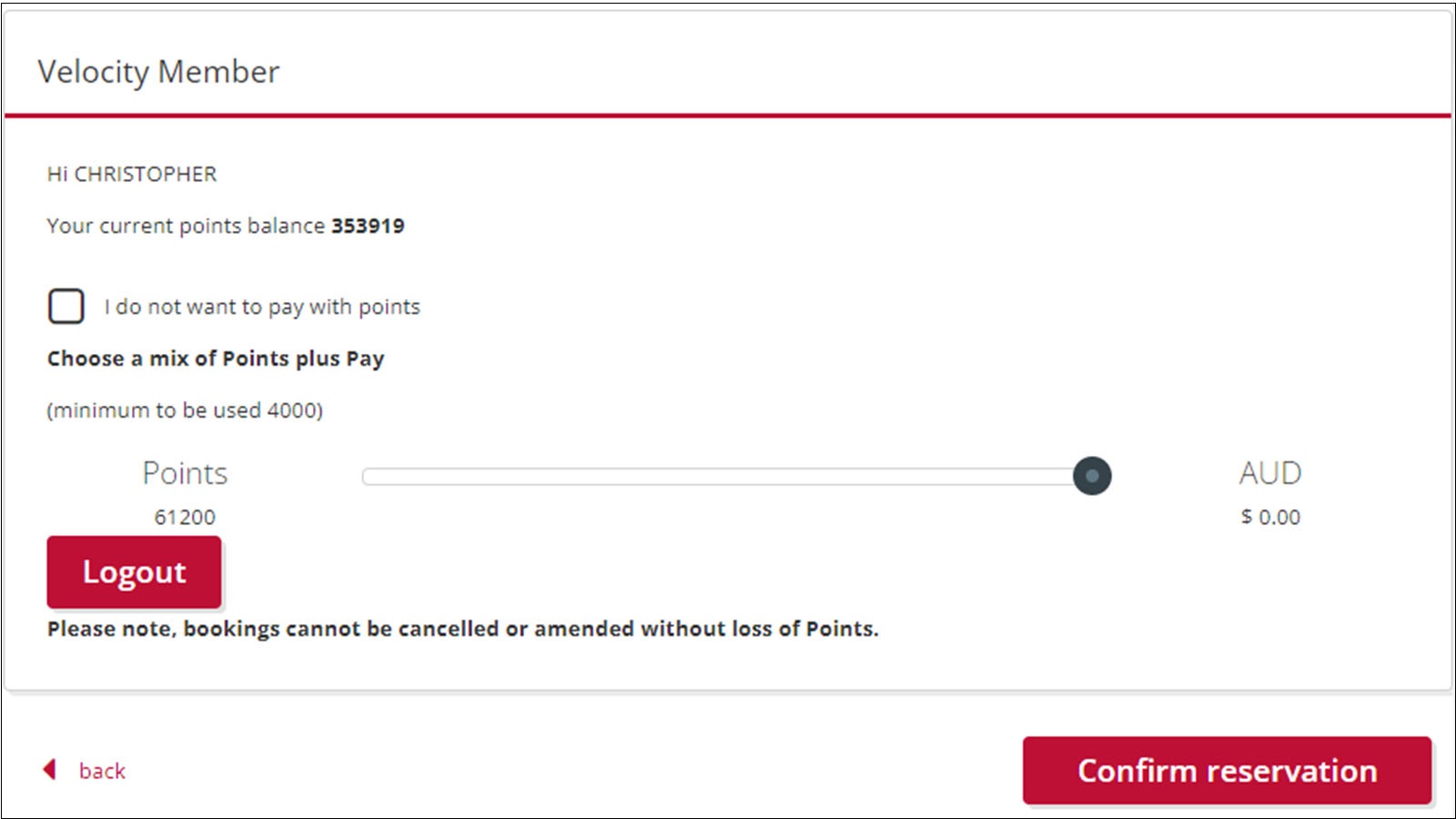Here is a detailed descriptive caption based on the image:

"This image depicts a section of a membership account information. The background is white, and at the top left corner, the header reads 'Velocity Member' in bold text. Directly beneath this header is a thin red line that extends horizontally across the top of the section. Below the red line, on the left side, there is a friendly greeting, 'Hi Christopher', followed by a statement of the current points balance, which is '353,919 points'.

Underneath this information is a rectangular box with a black outline. Inside the box, it reads, 'I do not want to pay with points', indicating that this option can be ticked to exclude points from being used for payment. 

Further down, there is a section titled 'Choose a mix of Points + Pay', with a stipulation stating 'Minimum to be used is 4,000 points'. Adjacent to this text is a slider, currently adjusted all the way to the right, showing a balance of 'AUD 0.00'. 

At the bottom of the section, there are two buttons; one is a 'Logout' button and the other is a 'Confirm Reservation' button."